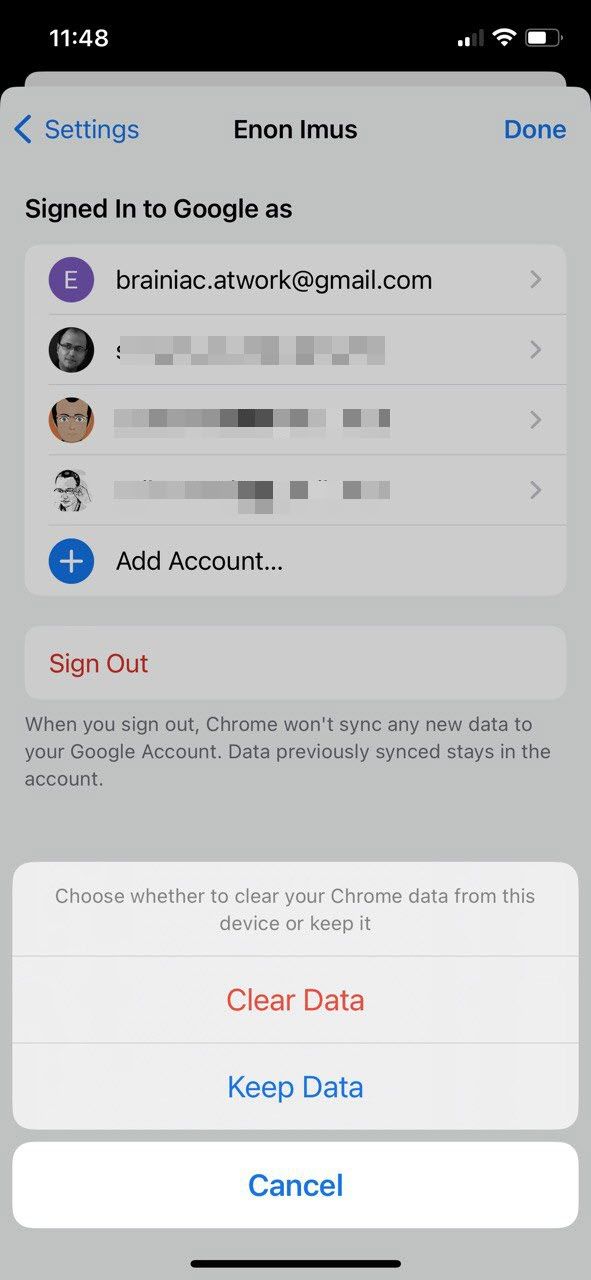The image displays a smartphone screen featuring an app page. At the top, the title "Anon Imoos" is visible, accompanied by a blue icon on the right side. Below this header, the settings option is highlighted in blue with the text indicating "Signed in to Google Ads."

The screen shows the first account, breniac.network.gmail.com, with its icon on the left side represented as a purple circle containing a white segment. Three email accounts are listed, but the email addresses are obscured with a mosaic effect to protect personal information.

Near the bottom, there is an option to "Add account," symbolized by a button with a blue circle and a white plus sign. Beneath this, the "Sign out" option is displayed in red text. A note explains that signing out will stop Chrome from syncing new data to the Google account, although previously synced data will remain in the account.

At the very bottom, a pop-up prompts the user to choose whether to clear Chrome data from the device or to keep it. This pop-up features three buttons: "Clear data" in red text, "Keep data" in blue text, and "Cancel" in blue text, arranged vertically.

This detailed description captures the structure and contents of the app page on the smartphone screen.